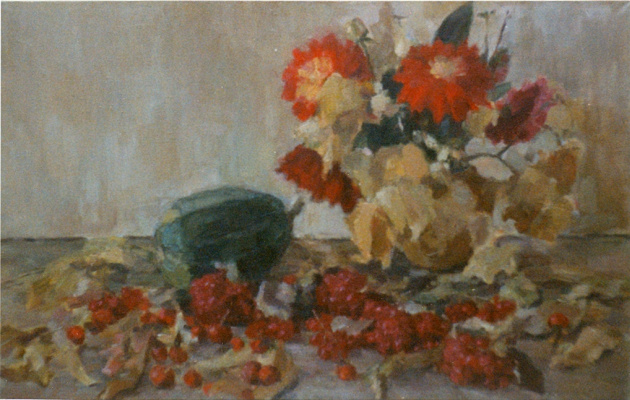The painting depicts an autumnal still life arrangement set against a beech-colored wall and a brownish wooden floor. At the center, slightly to the right, sits a gold vase brimming with a vibrant bouquet of red, yellow, and white flowers, complemented by interspersed green and brown leaves. To the left of the vase, a small green pumpkin adds an additional touch of rustic charm. Scattered at the base of the arrangement are various red berries, possibly cranberries or cherries, lying amongst brown leaves that evoke the essence of autumn. The overall composition, rendered in an artistic oil painting style, exudes a warm, seasonal feel with a rich palette of tan, brown, cream, red, yellow, green, and touches of off-blue, capturing the cozy, nostalgic atmosphere of an indoor autumn setting.